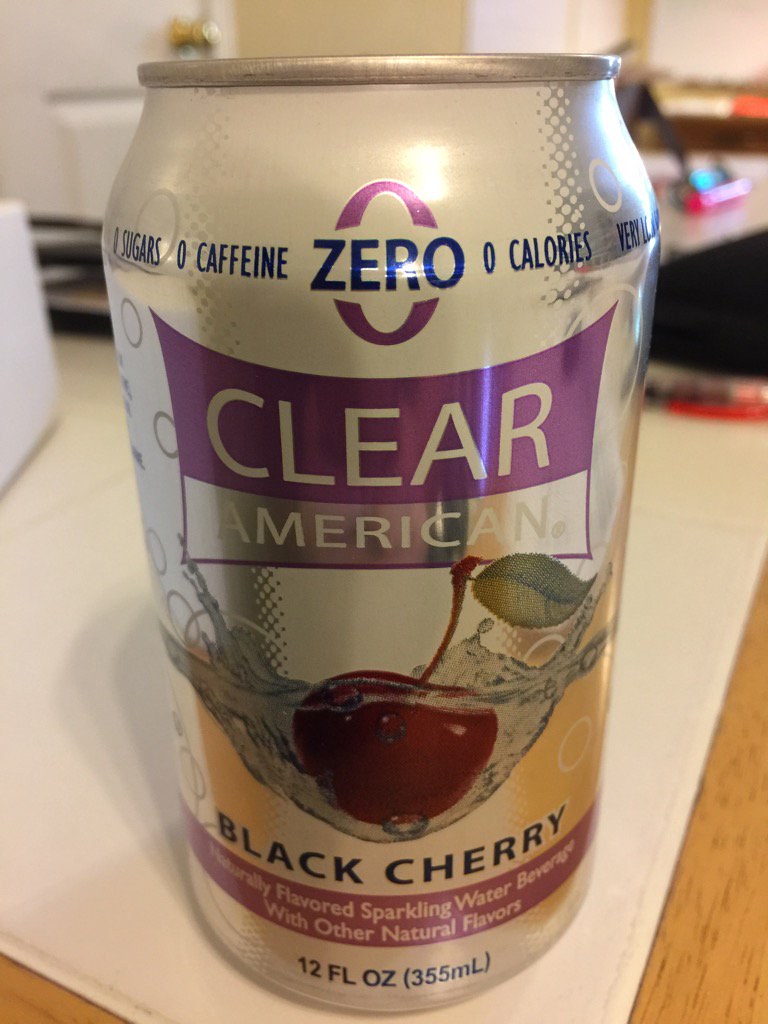The close-up image depicts a can of Clear American Black Cherry sparkling water positioned on a light brown wooden table. The can is set atop a thick, fuzzy white cloth with visible stitching. The can itself is aluminum with a silver finish and prominent labeling. At the top of the can in blue text, the word "ZERO" is flanked by two purple arches, and adjacent to it, the phrases "zero sugars," "zero caffeine," and "zero calories" are clearly written in blue. A bold purple banner in the middle features the word "CLEAR" in white text, and directly below it, "AMERICAN" is displayed on a smaller silver banner trimmed in purple. The label includes an image of a dark cherry with a stem and leaf, seemingly bouncing in water with splashes around it. Below the cherry, "black cherry" is printed in black text. Further down, the phrase "naturally flavored sparkling water beverage with other natural flavors" appears in white text on a thin red-pink strip. Additionally, the net weight "12 FL OZ (355 ml)" is stated in black text at the bottom. The blurred background reveals miscellaneous household items, adding context to the setting. The photo, likely taken on a phone, captures the can casting a shadow on the cloth, emphasizing the detailed design and vibrant colors of the product labels.